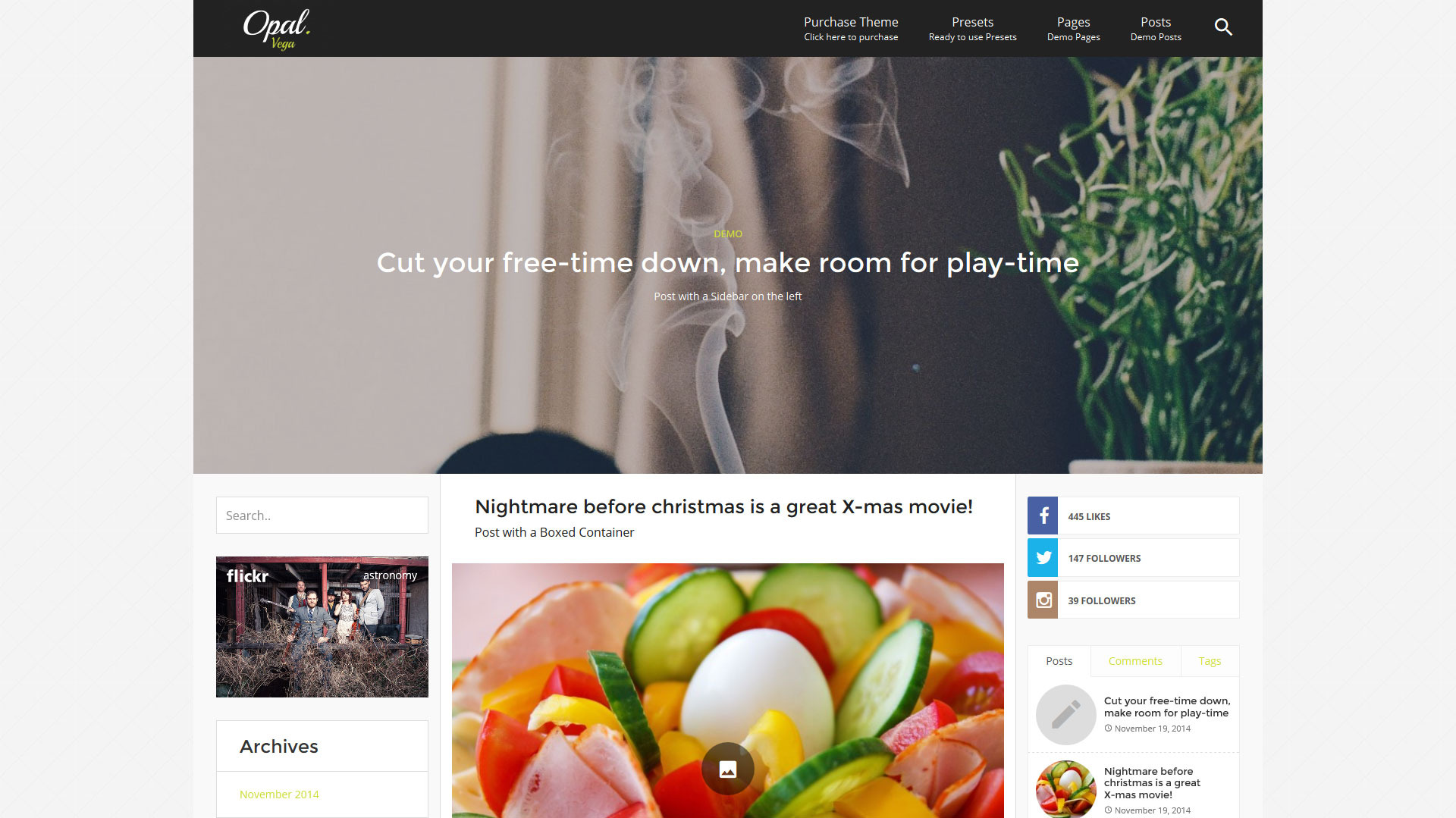This horizontally-oriented image features a screenshot with a very light gray background. Dominating the center top of the image is a horizontal box that contains a photograph of a plant accompanied by a plume of smoke in its center. Above this image, a black banner prominently displays the word "opal" in white text at the left-hand corner. Overlaid on the photograph in white text is the message: "Cut your free time down, make room for play time." The black banner also includes navigational sections labeled "Purchase Theme," "Presets," "Pages," and "Posts."

At the bottom portion of the image, there's a photograph of a salad dish garnished with various vegetables and a centerpiece egg. Above this photo, a text section reads: "Nightmare Before Christmas is a great X-mas movie," enclosed within a boxed container. To the left of this section, there's a search bar featuring the word "Flickr" and a label for "Archives" below it.

Towards the bottom right, social media icons for Facebook, Twitter, and another icon in brown with a white square are displayed. Under this area, textual snippets read: "Posts," "Cut your free time down, make room for play time," and "Nightmare Before Christmas is a great X-mas movie."